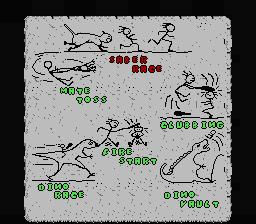The image is a full-color illustration centered on a splotchy white piece of paper. The paper is framed by a black border, although the border is thinner at the bottom. The edges of the paper have an artificially ragged look, suggesting it was altered by a computer.

At the top of the page, a short, straight black line serves as a divider. Above this line, a simplistic stick figure drawing depicts a cat chasing two people, all rendered in black ink. Below the line, there is a segment of red text, which is too small or unclear to be legible. 

Further down the page, another scene unfolds: a stick figure appears to have fallen flat, and beneath this figure is a line of green text, also illegible. Following this scene, another dividing line leads to additional stick figures; one is jumping up and hitting another figure on the head. Towards the bottom of the page is a crude rendition of a stick-figure dinosaur, accompanied by another person who is running and hitting someone on the head. 

The entire composition suggests a narrative or sequence of events, possibly from a computer game, though its exact purpose remains unclear.